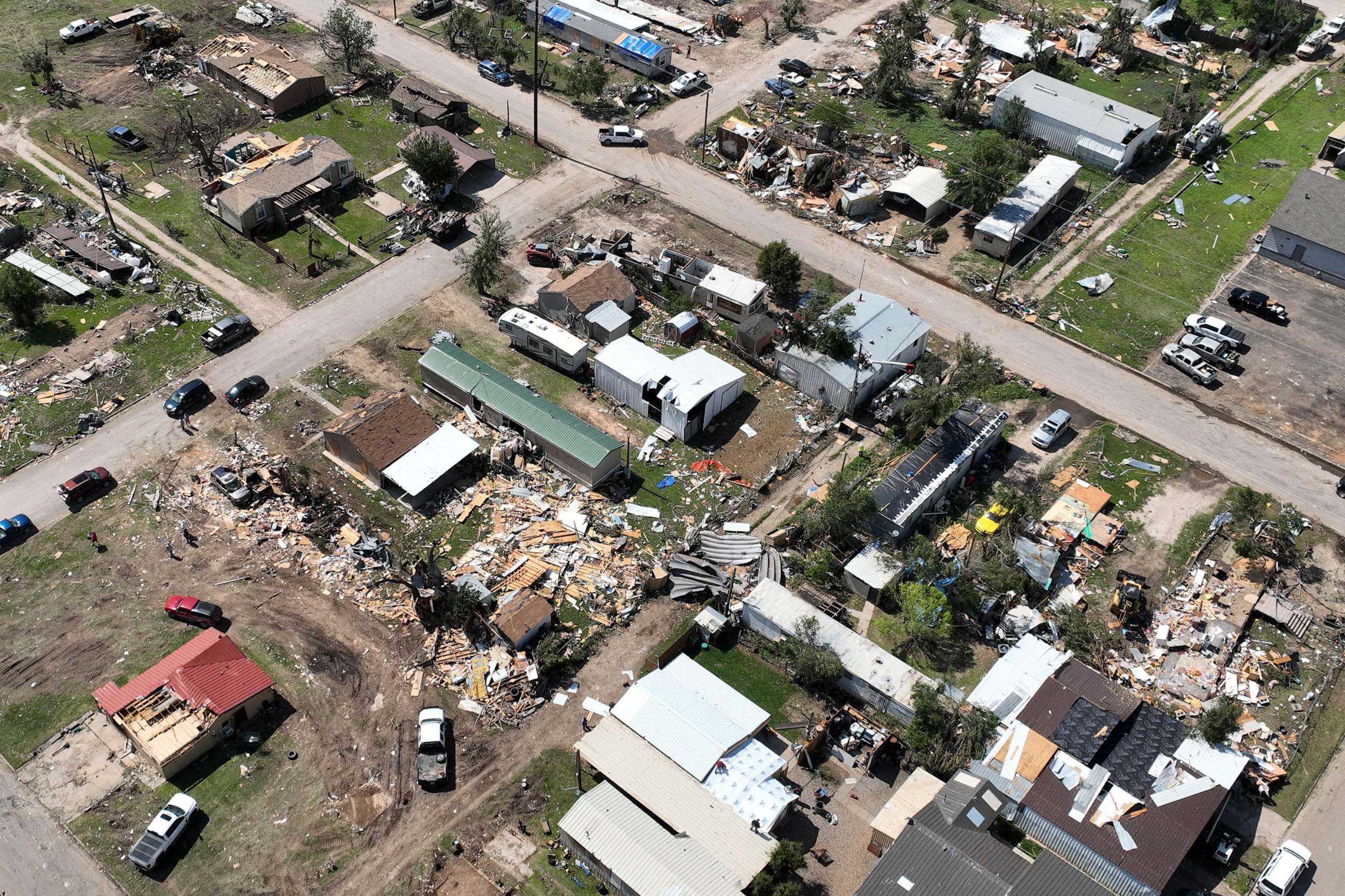This aerial photograph captures the extensive devastation wreaked by a tornado on a semi-rural town. The image reveals a vast swath of destruction stretching across multiple blocks, showcasing the stark contrast between intact and obliterated structures. Two main roads intersect the scene, along with several smaller streets, surrounded by parking lots, grassy areas, trees, businesses, and homes. 

Some homes appear relatively unscathed, with a fifth wheel trailer miraculously intact, while just across a gravel road, a nearby building is reduced to rubble and debris. Another house has its roof peeled off, exposing the interior. The image is strewn with wood, shattered concrete, displaced cars, and fragments of lives overturned. Concrete steps stand forlornly where a house once stood, emphasizing the sheer power of the storm. 

The photograph serves as a sobering assessment, illustrating the harrowing impact of the storm with debris scattered across the entire area and plots of land laid bare. The scope of destruction and the presence of green lawns and gray streets bespeak a neighborhood ripped apart, a poignant testament to the chaos wrought by the tornado.